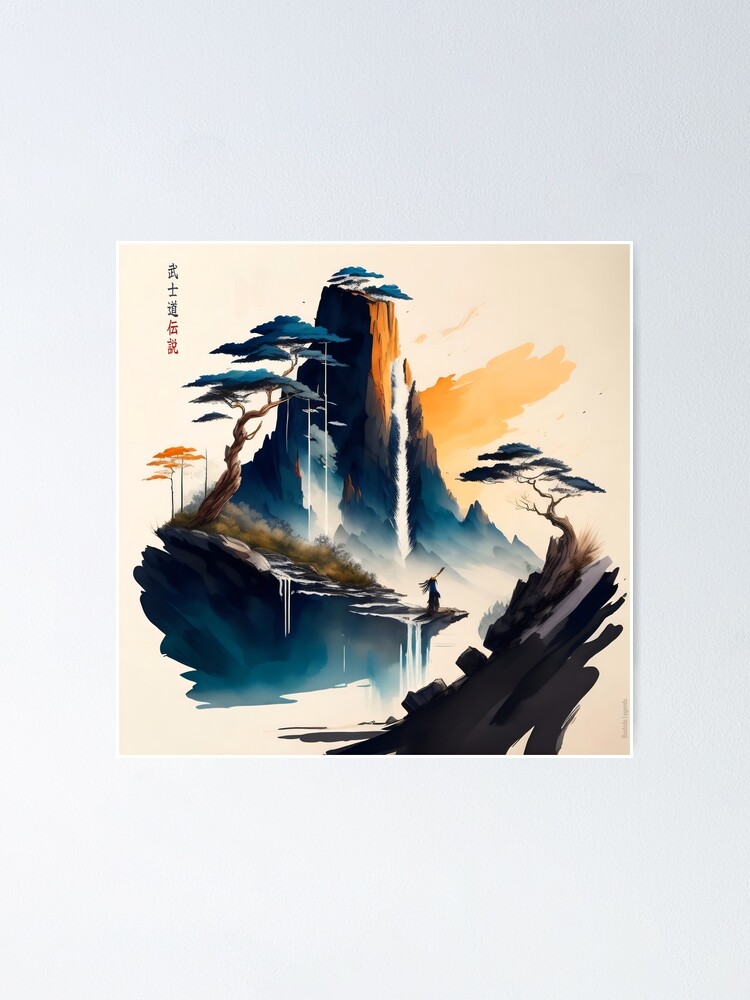The image depicts a Japanese-style painting set against a very light gray to white background. Dominating the center is a square with a thin white border. Inside this square, a minimalist yet evocative portrayal of a mountain, possibly Mount Fuji, is rendered in hues of orange, blue, and white. The background of the painting is a pale yellow.

To the left of the mountain, a tall, winding bonsai-like tree with green leaves rises gracefully. Adjacent to this tree, there is an inscription in black and red ink running vertically, featuring Japanese characters. At the base of the mountain, a tiny silhouette of a person can be seen, holding a rod aloft, adding a human element to the otherwise serene landscape.

On the right side of the painting, a cliff is depicted with another tree sprouting, its brown trunk supporting a tuft of green leaves at the top. The entire composition, with its floating elements and minimalist style, evokes a sense of tranquility and introspection.